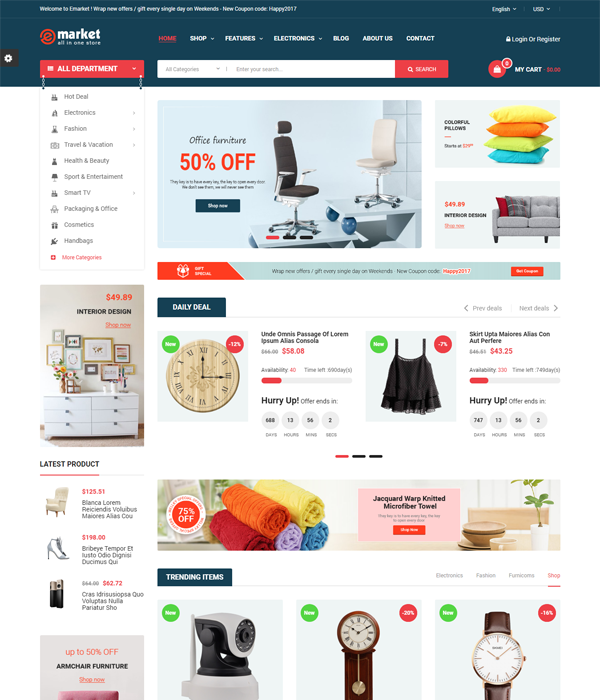**Website Layout: Detailed Description**

The image depicts a webpage of an online marketplace. The website’s name is "Market All-in-One Store," though the resolution of the image is noticeably poor. The page welcomes visitors with a tagline, “Welcome to the Market,” followed by an announcement about new offers and daily gifts, particularly highlighting special coupons on weekends. One such coupon code referenced is “HAPPY2877,” although the full accuracy of this code is uncertain due to the clarity of the image. This welcome text is presented in white on the left side of the page.

On the top right corner, there are options for setting the language to English via a drop-down menu, and the currency can be set to USD through another drop-down. Beneath these settings, the market's name appears again in red, while the phrase "all-in-one store" is displayed in white. 

Directly under this section is a navigation bar with the following options:
- Home (with a drop-down menu)
- Shop (with a drop-down menu)
- Features (with a drop-down menu)
- Electronics (with a drop-down menu)
- About Us
- Contact

Additionally, there is a login or register prompt on the right side of the navigation bar.

Below the navigation bar, there is an “All Departments” drop-down menu that is shown as opened. Adjacent to this is a search bar labeled “All Categories” where users can enter their search queries, accompanied by a red search button.

To the far right of the search bar is a shopping cart icon indicating “My Cart: $0.00” with a drop-down menu. This drop-down includes various categories such as:
- Hot Deals
- Electronics
- Fashion
- Travel & Vacation
- Health & Beauty
- Sport & Entertainment
- Smart TV Packages & Office
- Cosmetics
- Handbags

Moreover, there is a red link titled "More Categories" for additional browsing options.